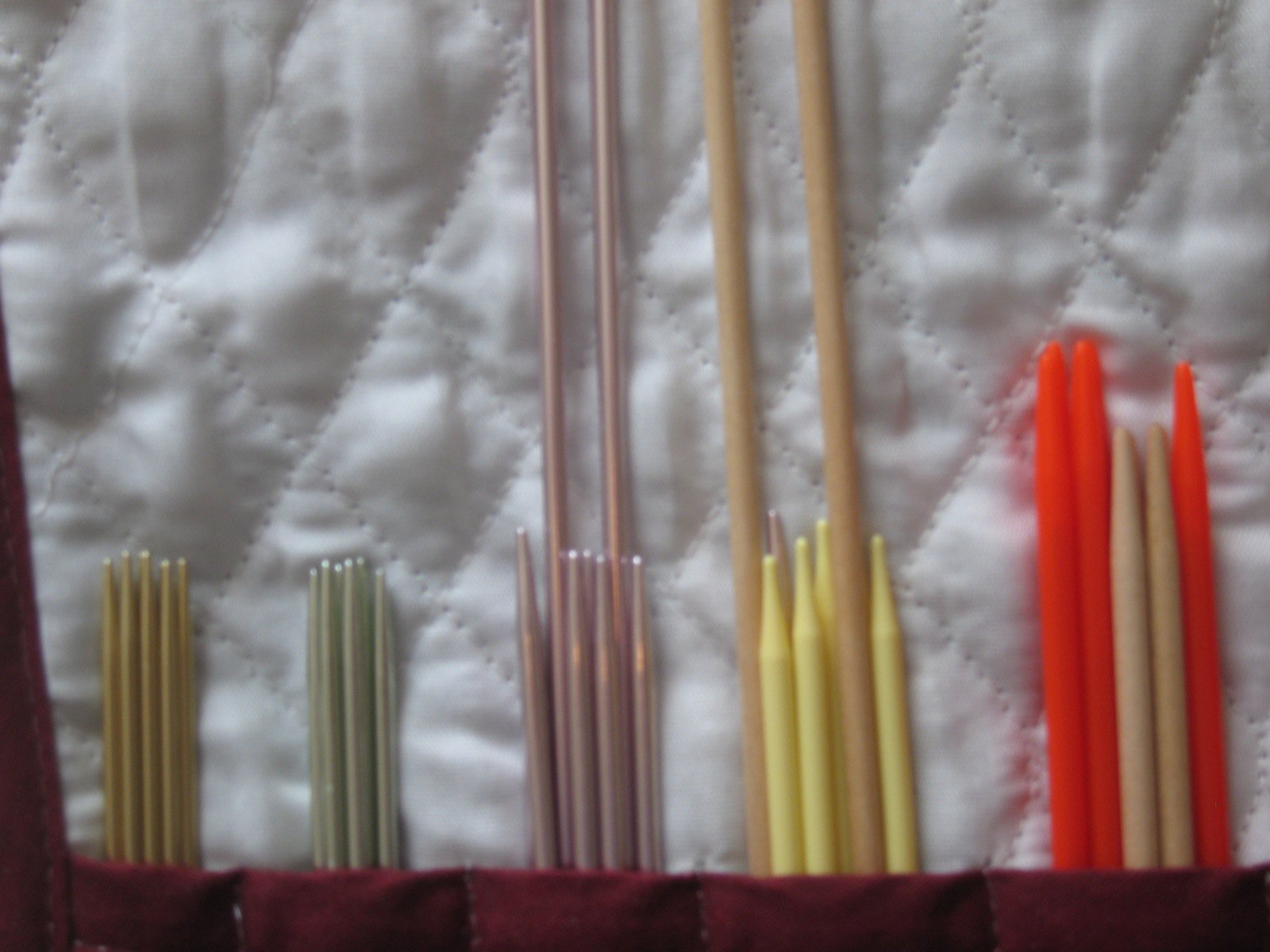The image portrays a neatly organized array of knitting needles in various colors and lengths, housed in individual pockets on a crocheted or quilted holder with a white background. The needles appear to be sorted into piles based on color, with groupings including silver, gold, metallic pink, metallic green, yellow, red, and natural wood hues. Notably, each color grouping features both uniformly sized needles and longer ones, and the rightmost section is a mix of red and tan/brown needles. The meticulous arrangement and the diverse metallic tones of the needles suggest a vibrant and organized knitting setup.